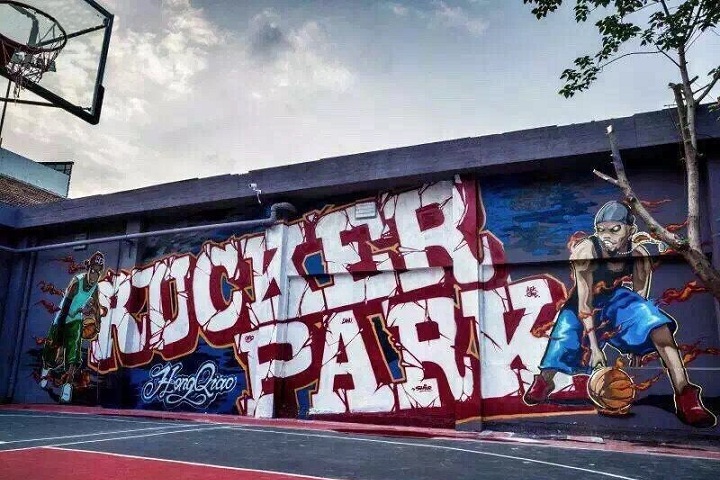The image depicts a vibrant scene at a basketball court adjacent to a building adorned with a commissioned mural. The court features a hoop with a clear backboard encased in a black frame, positioned in the upper left. The net, slightly worn, hangs from the hoop. The court below is painted in a dark navy blue with white lines and a red center. The backdrop of the scene is a grayish wall with a flat roof, connected on the left to a brick structure. Prominently displayed across this wall is a mural with the words "Rucker Park" written in white letters with a red shadow, set diagonally across a purplish background. This mural includes illustrations of street basketball players: on the left, a player with a teal tank top and green shorts dribbles a basketball, while on the right, another player, in a black tank top and blue shorts, executes a between-the-legs dribble. A small tree to the right of the wall adds a touch of nature, and the sky above is a mix of light blue and white clouds. A signature in cursive can be found at the bottom left of the mural, completing the artwork.